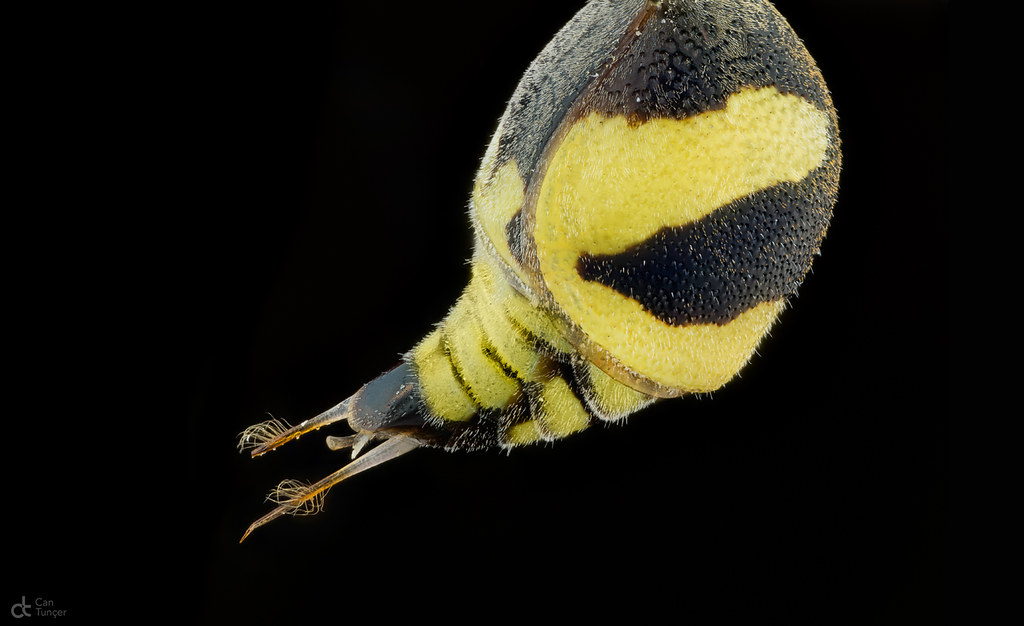This highly detailed and stylized close-up image showcases an unidentified insect or possibly a snail with distinct yellow and black coloration. The creature exhibits a pattern reminiscent of a bumblebee, with alternating yellow and black stripes. Its body is covered in fuzzy, hair-like structures, likely providing protection, and it features two prominent antennae on its head. The high-resolution photograph emphasizes the intricate scales and fur of the subject, though no eyes are visible. The background is entirely black, creating a stark contrast that makes the insect—or snail—stand out. The downward-facing position of the creature suggests it might be suspended in water, enhancing the mysterious and intriguing nature of the image.